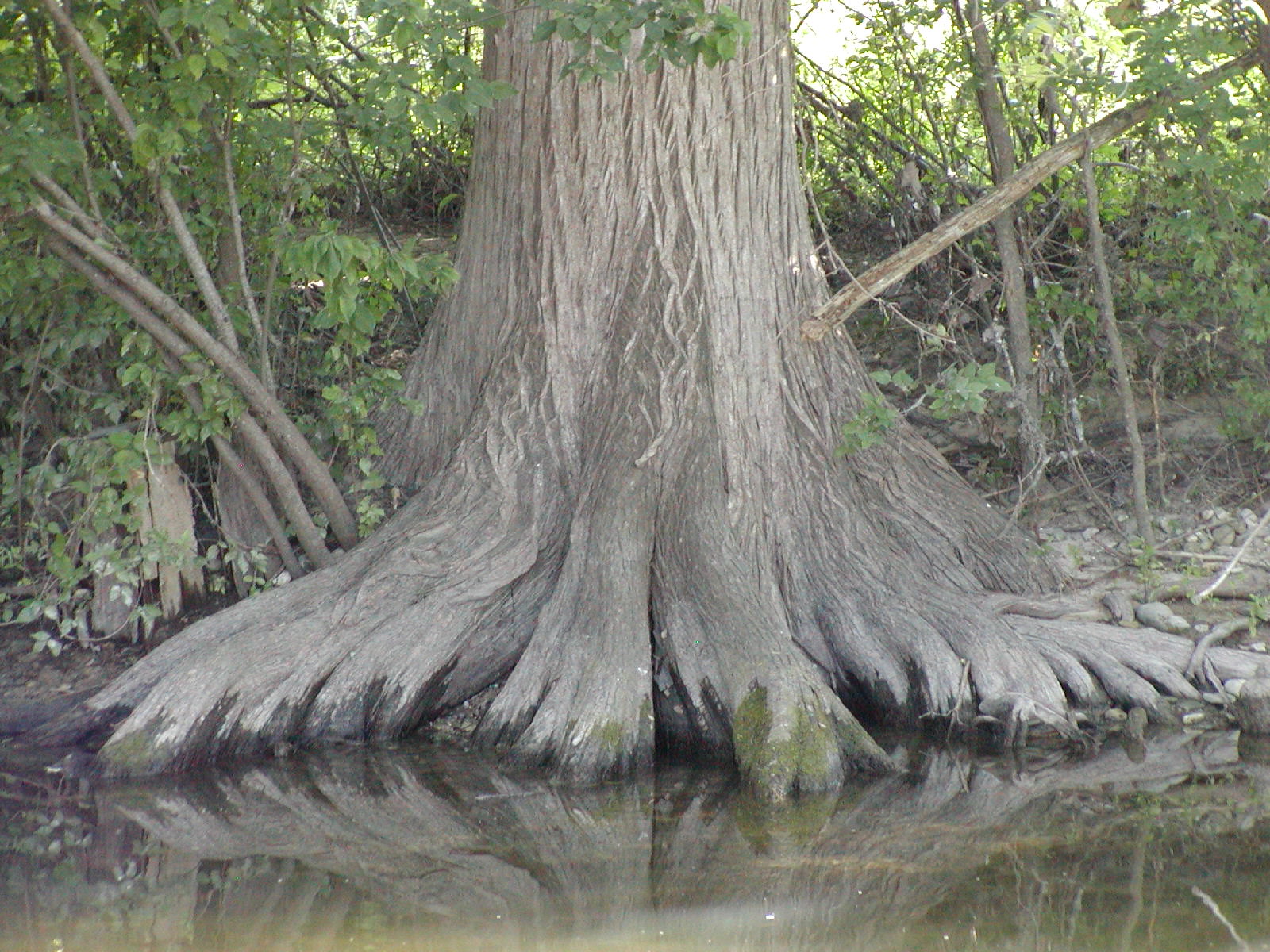The photograph captures a tranquil, natural scene featuring a very large, ancient tree situated in a swamp or waterway. The tree's massive, partially gray trunk dominates the center of the image, with its exposed roots extending into the smooth, tan-colored water in the foreground, creating a faint reflection. On the left side of the tree, smaller branches sprout, while the background is lush with various shrubs, smaller trees, leaves, sticks, and branches, adding a rich, green tapestry to the scene. Despite the overgrown appearance, the water's surface remains clear, contributing to the serene atmosphere, and there are no animals or inscriptions visible in the photograph.